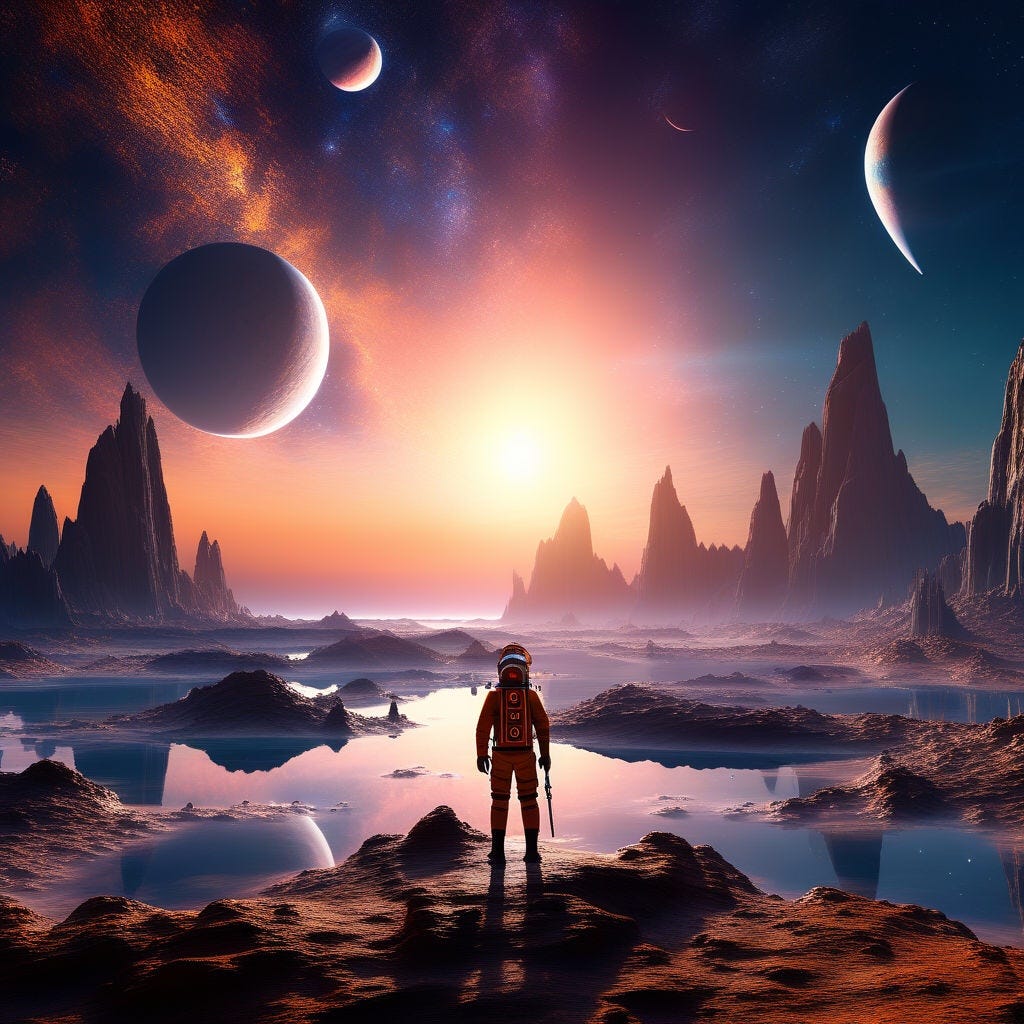The image presents a vividly detailed sci-fi scene featuring an astronaut clad in an orange suit with a helmet, standing on a rocky, extraterrestrial surface. The astronaut's back is turned towards the viewer, holding a long stick or object in their right hand, gazing out over the alien terrain. The ground beneath them consists of barren, rocky islands sporadically separated by patches of water or dirt, with tall, jagged mountains looming in the background. The landscape has puddles scattered throughout, creating reflections of the celestial features above. The sky is a stunning mix of blue hues with shades of orange and yellow, adorned with at least four distinct planets. These celestial bodies, alongside a distant sun and colorful galaxy dust clouds, create a surreal, otherworldly atmosphere. The entire scene is framed with a sense of vastness and exploration, capturing the wonder and isolation of space travel.